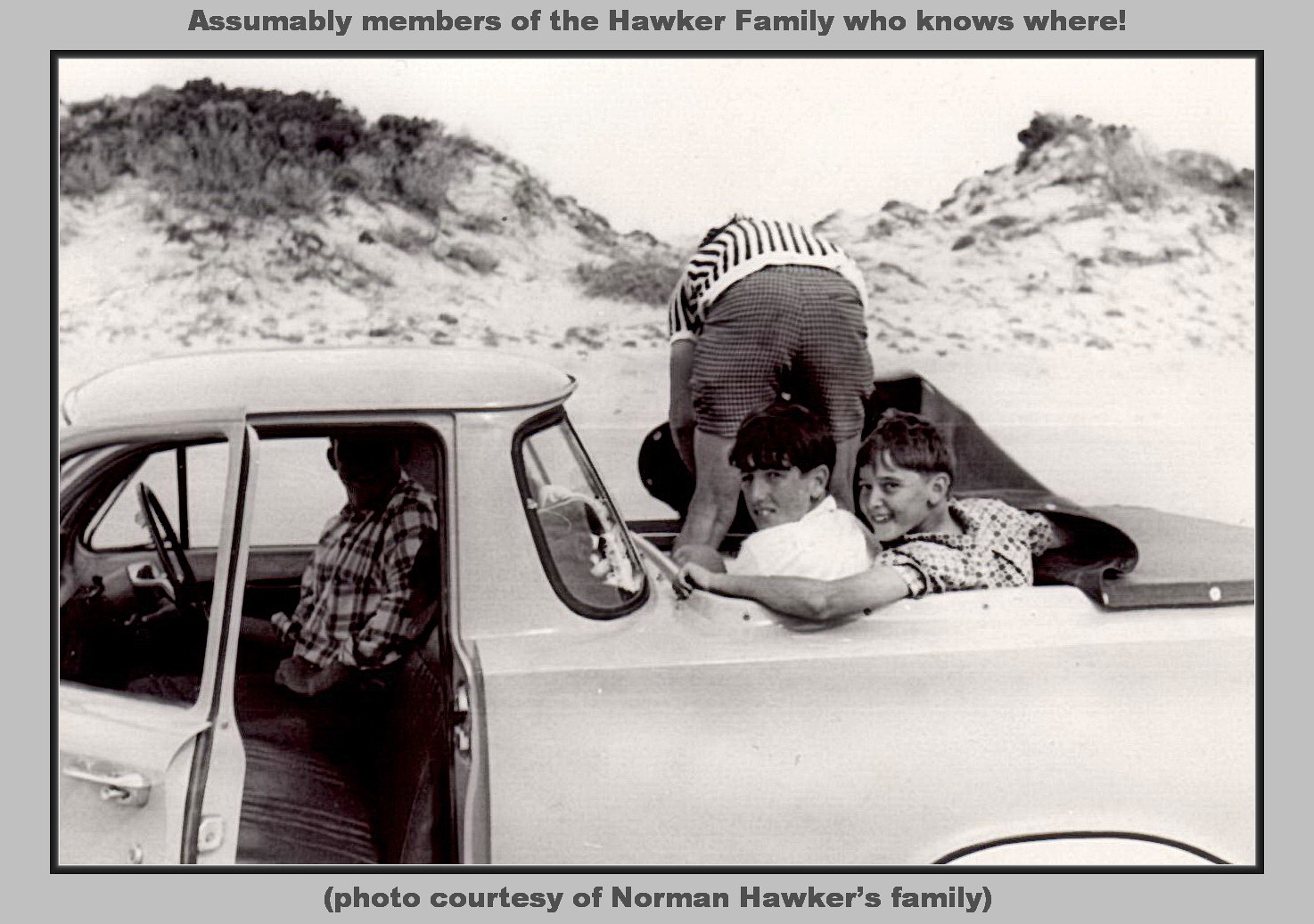This black-and-white photo features a vintage white pickup truck parked on the side of the road, with a backdrop of sand dunes or possibly mountains. The truck is distinguished by its snap-on black canvas cover over the back. In the front seat, a man with a checkered white shirt is seated behind the steering wheel on the right-hand side, with the passenger door open. In the open back of the truck, two boys in white shirts are smiling, and a woman in shorts and a white and blue striped shirt stands bent over near them. The photo is labeled at the top with the text: "Assumably members of the Hawker family, who knows where!" Below it, in parentheses, it reads: "Photo courtesy of Norman Hawker's family."